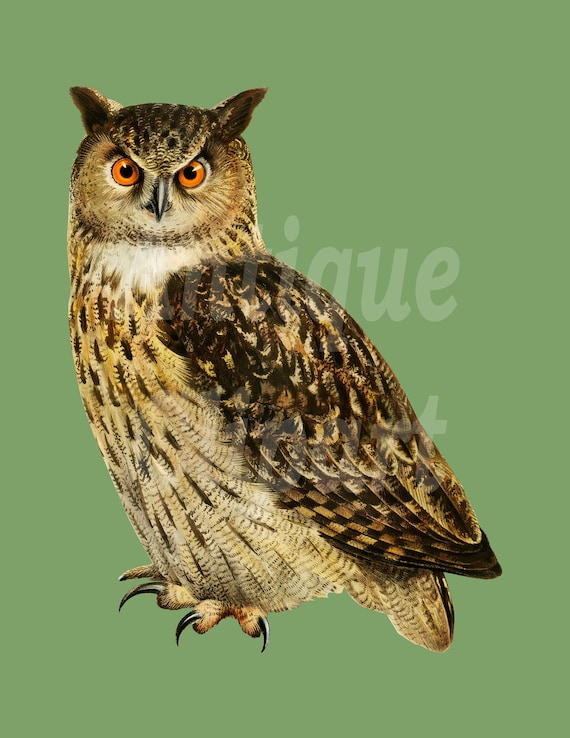This detailed image features a close-up view of a great horned owl with a digitally altered green background. The owl is prominently displayed in the center with its head turned towards the camera, appearing to scrutinize the viewer with its piercing, bright orange eyes. The owl's face forms a scowl-like expression, accentuated by the feather tufts mimicking ears atop its head. Its chest exhibits a yellowish-brown hue adorned with dark speckles, while its wings boast dark, brownish-black feathers. The owl's sharp talons and black beak add to its fierce appearance. There is a faint, two-word watermark diagonally superimposed over the image, with the first word decipherable as "Antique," although the second word remains unclear. The overall composition, coupled with the expression and detailed features of the owl, gives the image an intense and captivating aura.